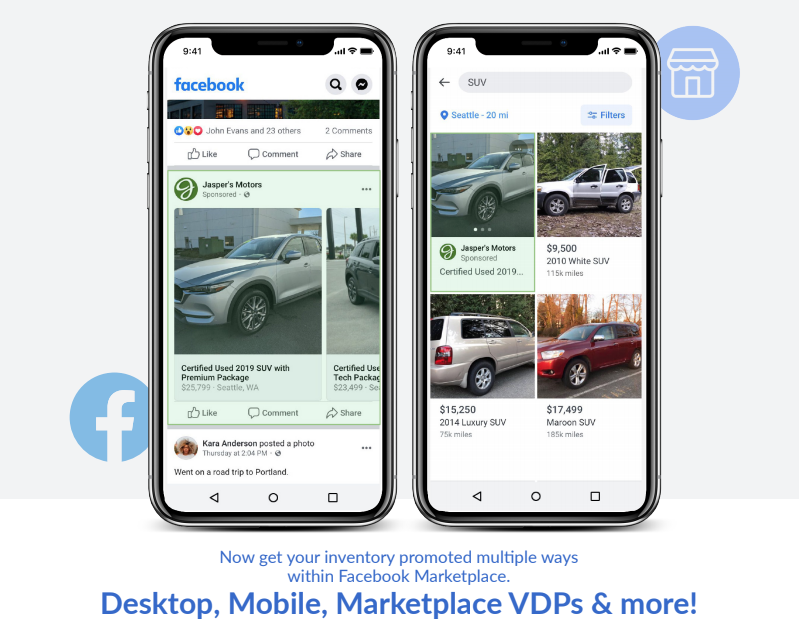The image depicts a detailed view of the Facebook Marketplace interface as seen on a smartphone, displayed in a side-by-side comparison of two different screens. 

In the top section of both screens, you can see the standard indicators for battery life, network connection strength, and the time, 9:41. The Facebook logo, presented in large blue letters, occupies the left side. A search bar is visible along with a notification icon represented by a gray circle containing a black circle and an embedded image. 

The first screen displays a post from "Jaspers Motors," labeled as sponsored content. In this post, there are images of two certified used cars—a silver 2019 SUV with a premium package priced at $25,799, and partially visible, another car listed for $23,499, both presumably located in Seattle, Washington. The post includes options for liking, commenting, and sharing. Further down, another post by Kara Anderson is visible, indicating she posted a photo from her road trip to Portland.

The second screen focuses on a search result page within Facebook Marketplace, where "SUV, Seattle" is typed into the search bar. The search results include multiple vehicle listings: the same silver SUV from Jaspers Motors, a 2010 white SUV for $9,500, a 2014 luxury SUV for $15,250, and a maroon SUV for $17,499. Each listing details the price, year, and mileage of the vehicles. Promotional text in blue encourages users to get their inventory promoted across various platforms within Facebook Marketplace.

In the background, the computer interface shows the familiar Facebook layout, with the Facebook "F" icon in the lower-left corner and the home button depicted in a periwinkle-colored circle situated at the top.

This detailed description captures the essence and functionality of the Facebook Marketplace as presented in the image.